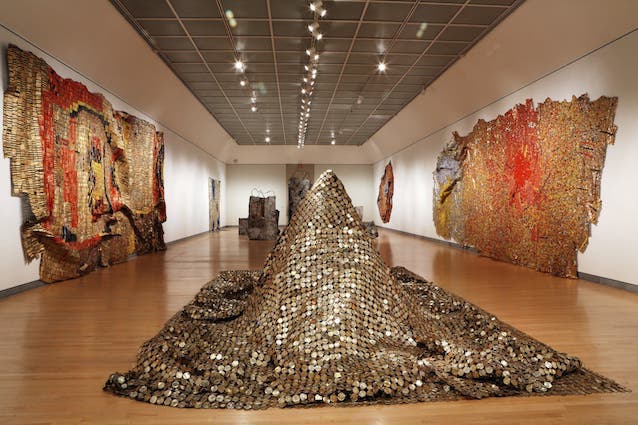The photograph captures an indoor scene that is likely within a museum or art gallery. The room is long and narrow with reflective wooden floors that add warmth to the environment. The walls, painted white, are adorned with various artifacts and artworks that include old cloths or materials stitched into large murals. These exhibits line both the left and right sides of the hallway, showcasing a myriad of colors and textures, particularly red, black, and gold.

At the center of the room stands a prominent, pointed structure draped in a gold-patterned cloth decorated with metallic circles, resembling a pyramid. This central piece is eye-catching, although its exact form beneath the cloth remains concealed. The ceiling is lined with gray tiles that house three rows of spotlights and fluorescent lights, effectively illuminating the entire space.

In the background, additional exhibits are visible, including what appears to be a rocky structure on the center-left side. The details are somewhat obscured due to the image's compression, but the overall ambiance and intricacy of the exhibits are clearly discernible. This detailed and well-lit display area provides a rich visual experience typical of a curated museum gallery.